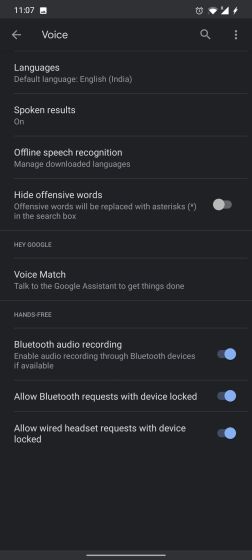This image depicts an iPhone screen showcasing the voice settings. The black screen features "Voice" prominently in white text at the top, with an arrow pointing to the left indicating a back navigation option. The status bar displays the current time and connection icons.

The voice settings menu includes the following options:

1. **Languages**: Shows the default language set to English (India).
2. **Spoken Results**: Enabled, providing spoken feedback for queries.
3. **Offline Speech Recognition**: Manage downloaded languages for offline use.
4. **Hide Offensive Words**: Disabled. Offensive words will not be replaced with asterisks in the search box.
5. **Hey Google**: Always on, enabling voice activation for the Google Assistant.
6. **Voice Match**: Allows the Google Assistant to recognize your voice to perform tasks.
7. **Hands-Free**: Standard settings without options to disable.
8. **Bluetooth Audio Recording**: Enabled, allowing audio recording through Bluetooth devices.
9. **Allow Bluetooth Requests with Device Locked**: Enabled, permitting Bluetooth requests even when the device is locked.
10. **Allow Wired Headset Requests with Device Locked**: Enabled, allowing wired headset requests when the device is locked.

The image effectively captures the detailed configuration options available in the voice settings of the iPhone.